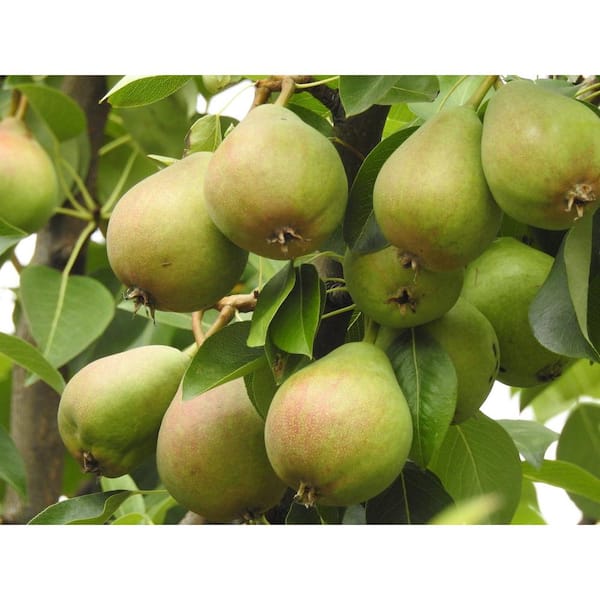This is an exceptionally detailed close-up photograph of a pear tree. The image showcases lush green leaves and their stems extending from the branches, with 11 pears hanging prominently. Each pear exhibits a light green hue with a slight brownish tint towards the bottom, and a few even have a touch of red, indicating varied ripeness. The pears are arranged in two distinct rows—six across the top and three at the bottom, with two partially concealed on the middle right. The green foliage nearly matches the color of the pears, and the background reveals small white spots, likely indicative of the sky. A large brown section of the tree trunk is also visible, adding to the naturalistic detail of the scene, all under daylight.